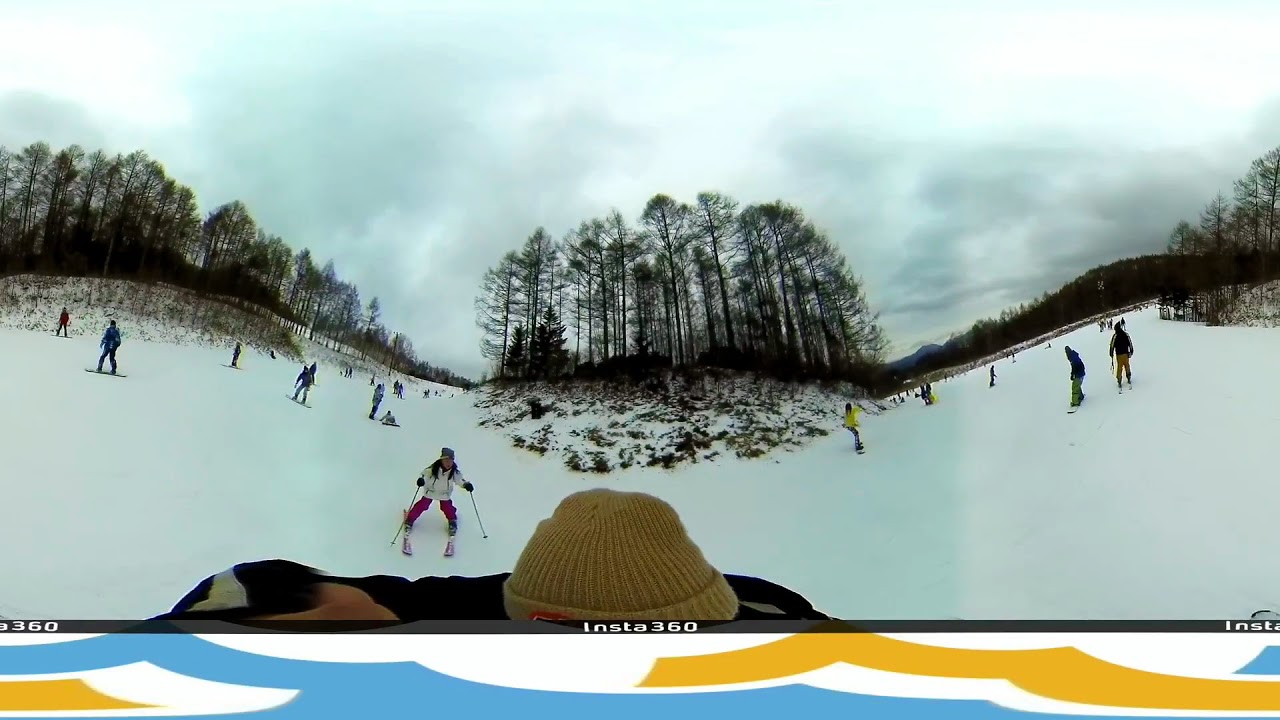The image depicts an expansive outdoor ski slope bustling with activity. At the forefront stands a skier, identifiable by her white jacket and red pants, confidently gripping her ski poles as she navigates the snowy landscape. Surrounding her, clusters of trees populate the scene, with some centrally located and others flanking both sides of the hill. The terrain, mostly blanketed in snow, reveals patches of grass peeking through in areas where the cover is thin. 

In the bottom middle of the image, the mustard-colored knit cap of another skier, who is capturing this 360-degree view, is prominently visible along with the black top they are wearing. This perspective indicates that most other skiers and snowboarders are descending the slope towards the camera. The hill ascends behind this skier and slopes downward in front, showcasing around twenty individuals on the left and right sides, their small outlines suggesting a diverse crowd of skiing and snowboarding enthusiasts. 

Despite their tiny appearances, these figures animate the scene with dynamic movement, appearing to be a mix of beginners and intermediate skill levels. Overhead, the sky is overcast with gray clouds, enhancing the wintry atmosphere. Amidst the throng, a little girl clad in a white ski jacket and pink pants skis closely behind the main skier, adding a touch of youthful exuberance to the picturesque, bustling ski slope. The caption "Insta360" marks the image, connecting it to the perspective provided by the skier in the vibrant yellow cap.